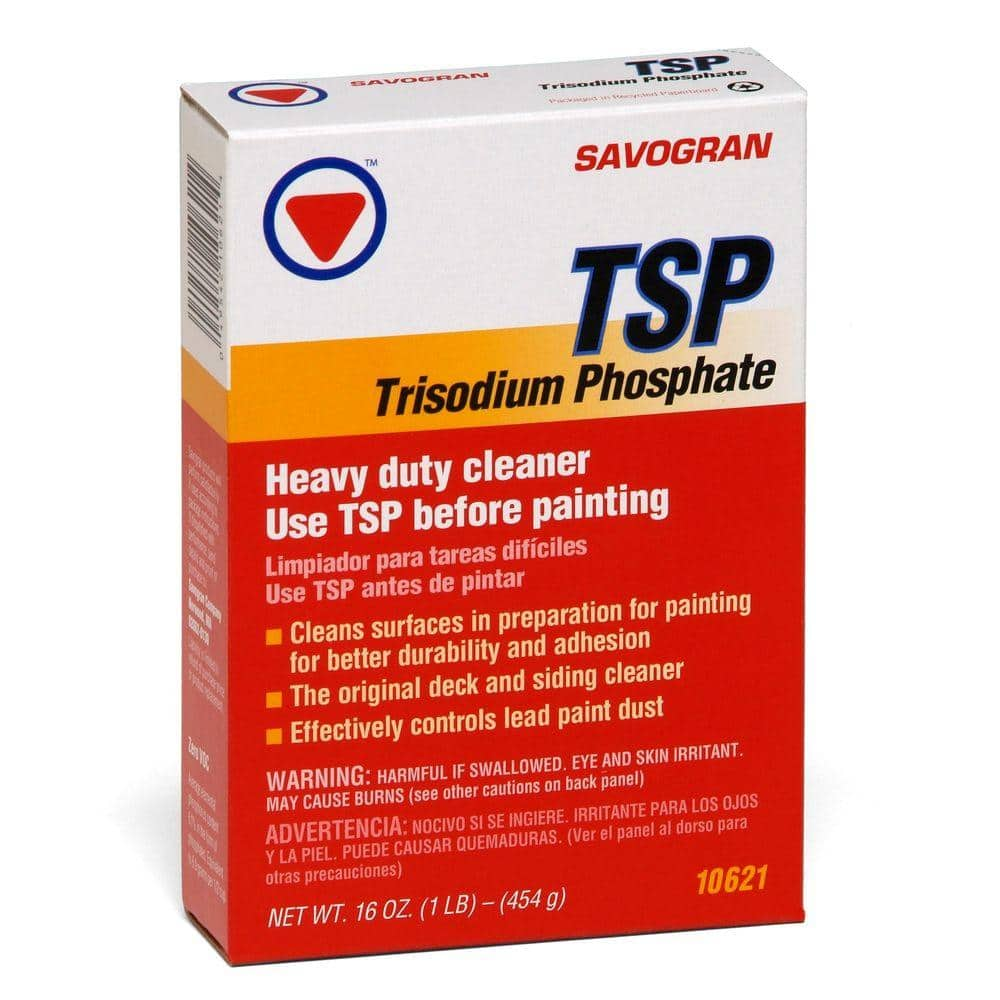This close-up image showcases a package of Trisodium Phosphate (TSP) from Sabogran, designed to be featured in an advertisement with a white backdrop. Dominating the image is the product itself, a white box accented by a dark red lower section. The top right of the package prominently displays the Sabogran logo in red. To the left, a blue circle contains a downward-pointing, red triangle, which is likely the company's symbol. 

Bold black letters spell out "TSP" on the front, with "trisodium phosphate" written just below. Within the red section, white text highlights its primary use: "Heavy-duty cleaner, use TSP before painting." This is followed by Spanish text: "Limpiador para tareas difíciles, use TSP antes de pintar." 

Further information is provided in yellowish-orange bullet points, explaining that the cleaner prepares surfaces for painting to enhance durability and adhesion and that it's effective for controlling lead paint dust on decks and siding. A warning at the bottom, in both English and Spanish, cautions that the product is harmful if swallowed and may irritate eyes and skin, with additional cautions listed on the back panel. The package also mentions that it contains 16 ounces (1 pound) of product. The left side of the box is partially visible, showing a barcode at the top with more descriptive text below.